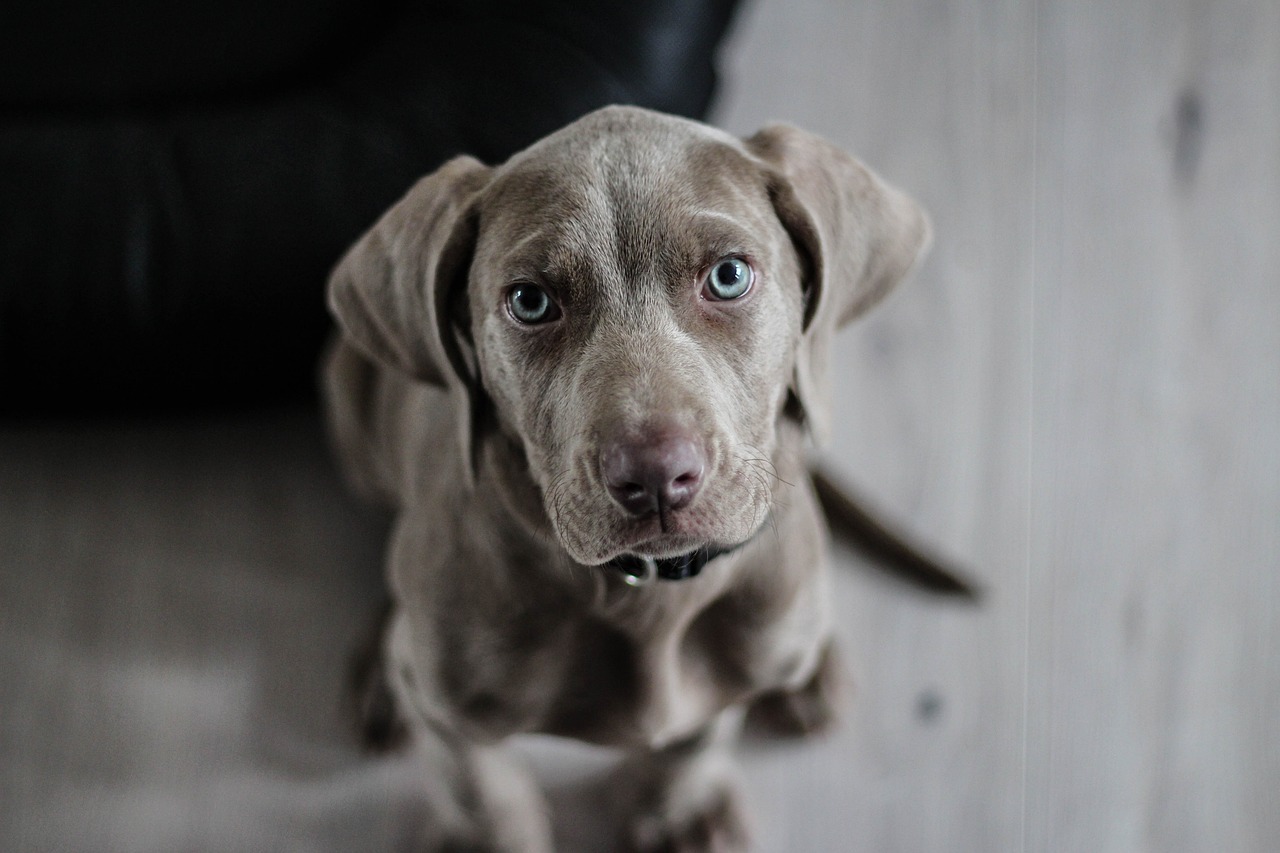This horizontally oriented, realistic photograph captures a young dog sitting on a hardwood floor. The background is split in color, with a light gray on the right and a darker gray on the left, though it remains blurry and indistinct. The floor beneath the dog features a subtle wood pattern. The central focus of the image is a young brown dog, likely either a chocolate Labrador Retriever, a Chesapeake Bay Retriever, or possibly a Weimaraner, characterized by its soft, sleek, grayish-brown fur, and distinct light blue eyes. The dog, which appears to be around six months to a year old, is sitting on its hind legs with its tail, hind legs, front legs, and chest all visible. It has a black collar adorned with a stainless steel ring. The dog looks directly up at the camera, which is pointed downwards at it, exhibiting a calm and placid expression. The photograph eloquently conveys the dog's serene demeanor, highlighting its healthy and soft appearance, which is invitingly pettable.